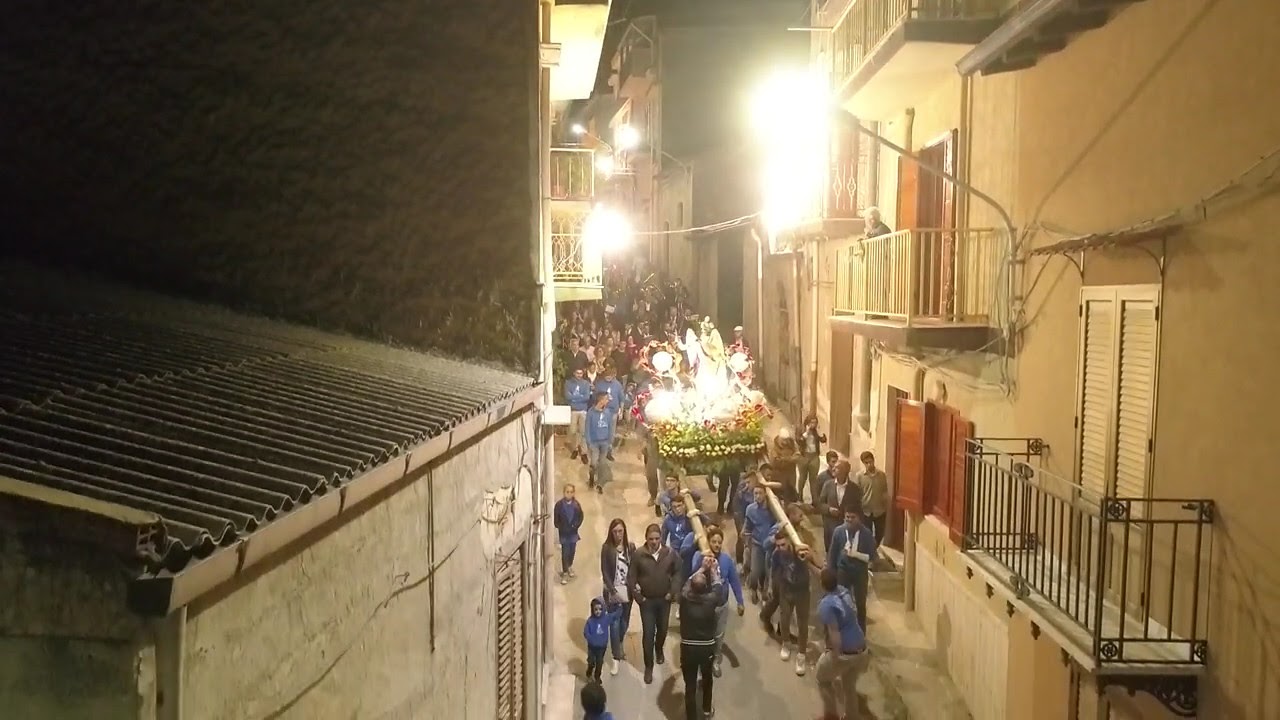The image depicts a bustling night-time festival on a narrow, sloped street lined with tall, tan, apartment buildings with balconies. The scene is illuminated by numerous lights. A large crowd is navigating down the alleyway, with a particular focus on a group of men dressed in blue. These men are carrying a prominent float, adorned with flowers and lights, on long wooden beams over their shoulders. The float features a green base, a statue, and two lighted spheres on top. Amidst the spectators, an elderly woman can be seen observing the event from a balcony on the right side. The buildings showcase a mix of white doors, shutters, and metal roofs, adding to the traditional ambiance. The entire atmosphere suggests a significant cultural or traditional celebration, possibly of Asian or Middle Eastern origin, given the attire and the ceremonial float.